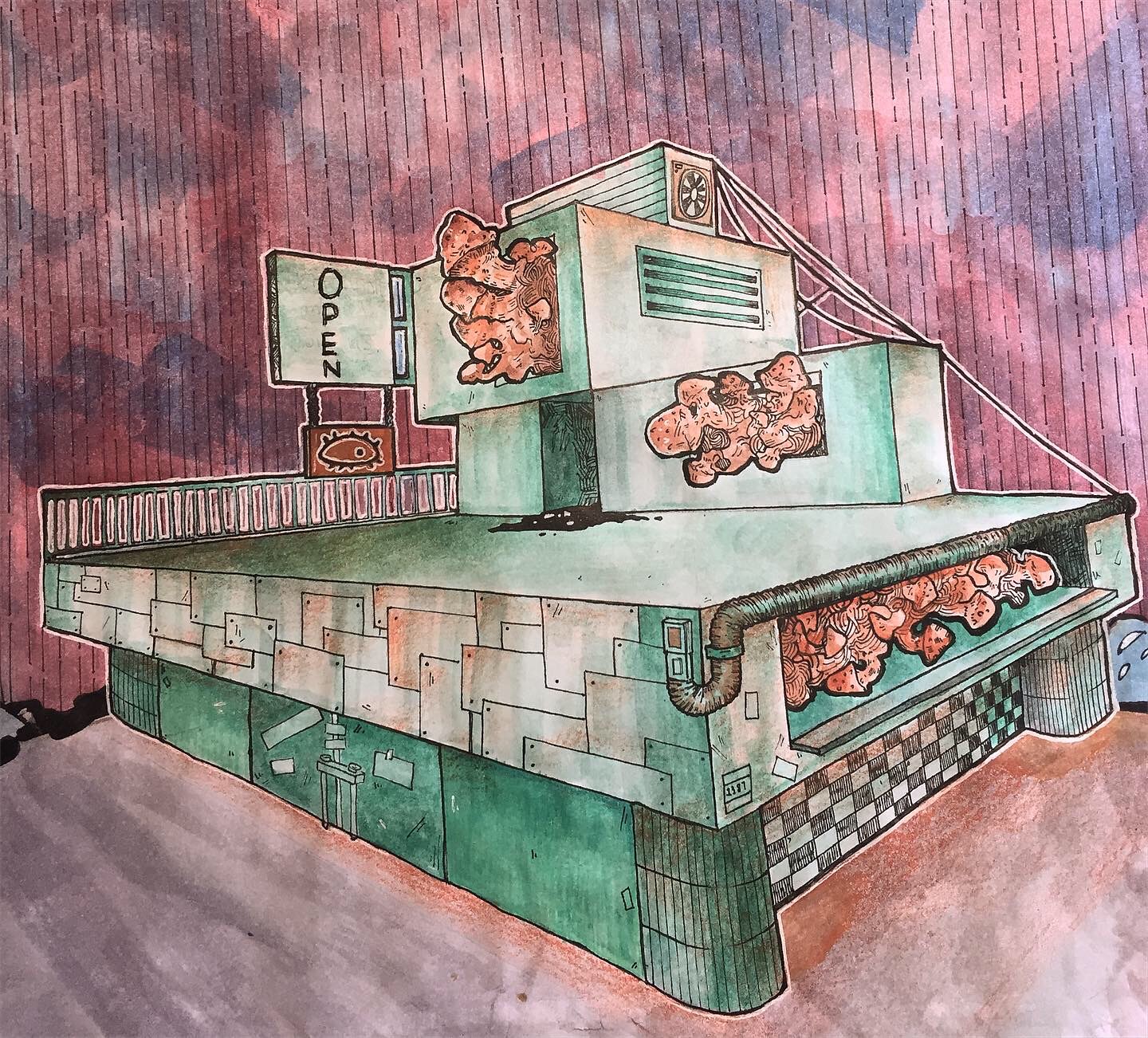This artwork is a vibrant and detailed watercolor painting, initially outlined in ink, of a somewhat abstract building. The artist has employed a captivating palette of light orange-red, deeper pink-red, navy blue-purple, medium green, and emerald green tones. The background melds pink-red and blue hues, creating a dynamic sky that frames the structure. The building itself stands out with its emerald green and light orange-red hues. Intriguingly, an "open" sign is depicted towards the top left corner, while whimsical elements like mushrooms appear to be protruding from its windows and doors. Additionally, there is a checkerboard pattern adorning the bottom right side, adding to the piece's unique charm and intricacy.